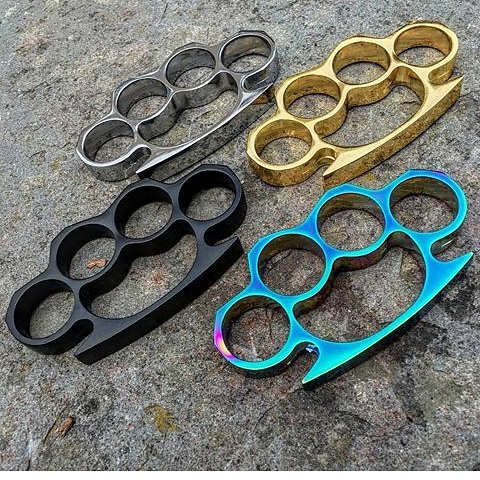This is an angled photograph of four pairs of brass knuckles, resting closely together on a dirt-embedded concrete surface. The brass knuckles are positioned with their middle sections facing the left corner and their bottoms angled toward the bottom right of the image. At the top sits a silver pair with some dark shading. Below it on the left is a black pair, and to the right of that, a golden pair. Closest to the camera at the bottom is a blue pair featuring a purple stripe and some yellow detailing on one side. The ground, grey with black and brown debris, suggests an outdoor setting.